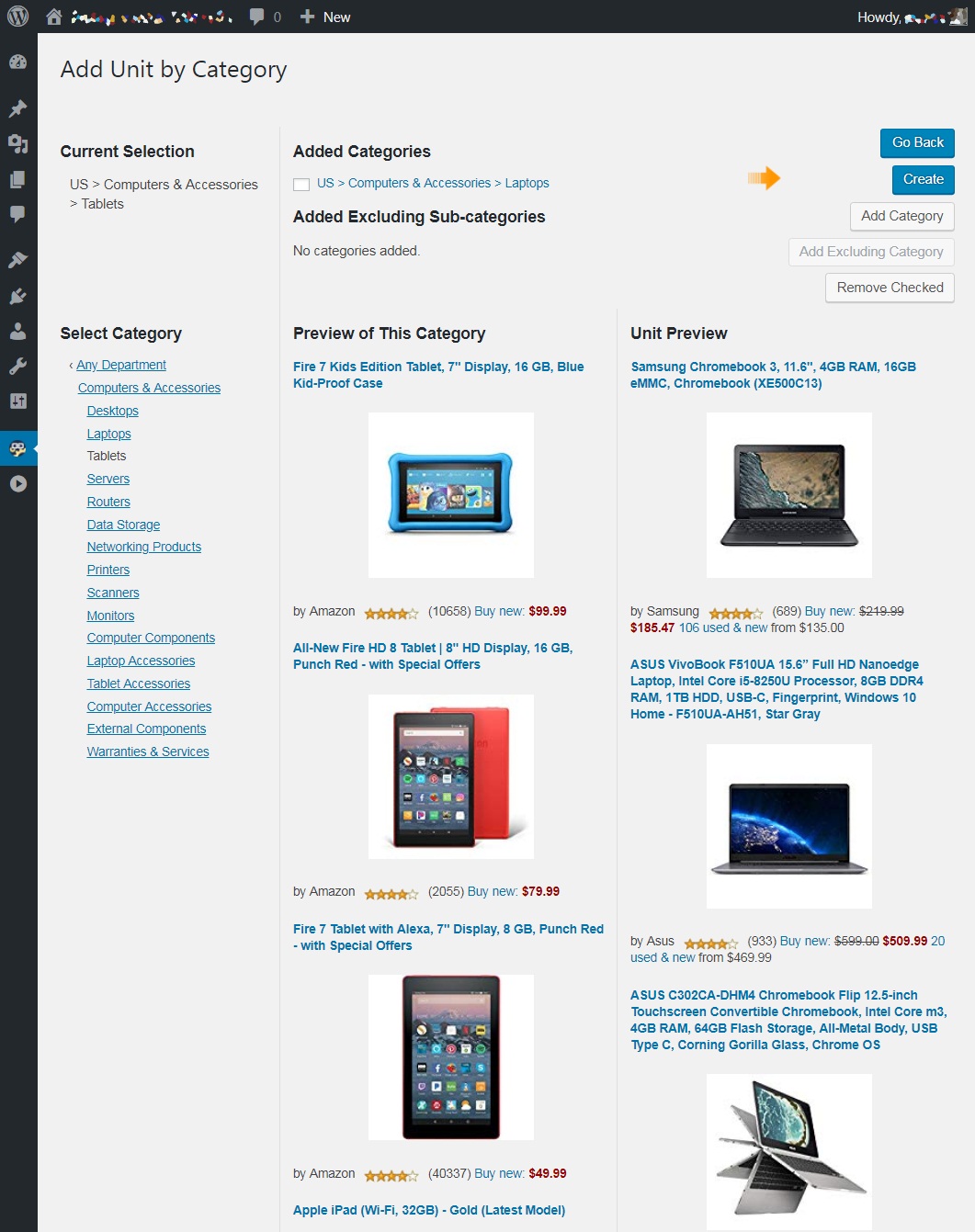The image showcases a PC application with a portrait orientation on a bluish off-white background. The interface is framed by thin menu bars on the left and top sides, populated with various icons. Although the icons are somewhat small, discernible figures include a thumbtack, pin, person, and wrench, among other common application icons.

At the top of the screen, there are several white squiggly lines on a black background, which appear to be notifications or system statuses that are not easily readable. The main section of the application prominently displays the title "Add Unit by Category." Below this title are subheadings labeled "Current Selection," "Added Categories," and "Added Excluding Subcategories."

To the right of these subheadings are several buttons. Blue buttons labeled "Go Back" and "Create" are clearly active, while gray buttons offer options like "Add Category" and "Remove Checked." There is also a grayed-out button for "Add Excluding Category," indicating this option is currently inactive.

Beneath the buttons, there is a grid layout displaying six visible tech items, specifically tablets and laptops. Each item is paired with blue hyperlinks for additional information, allowing the user to click and explore further details about each product.